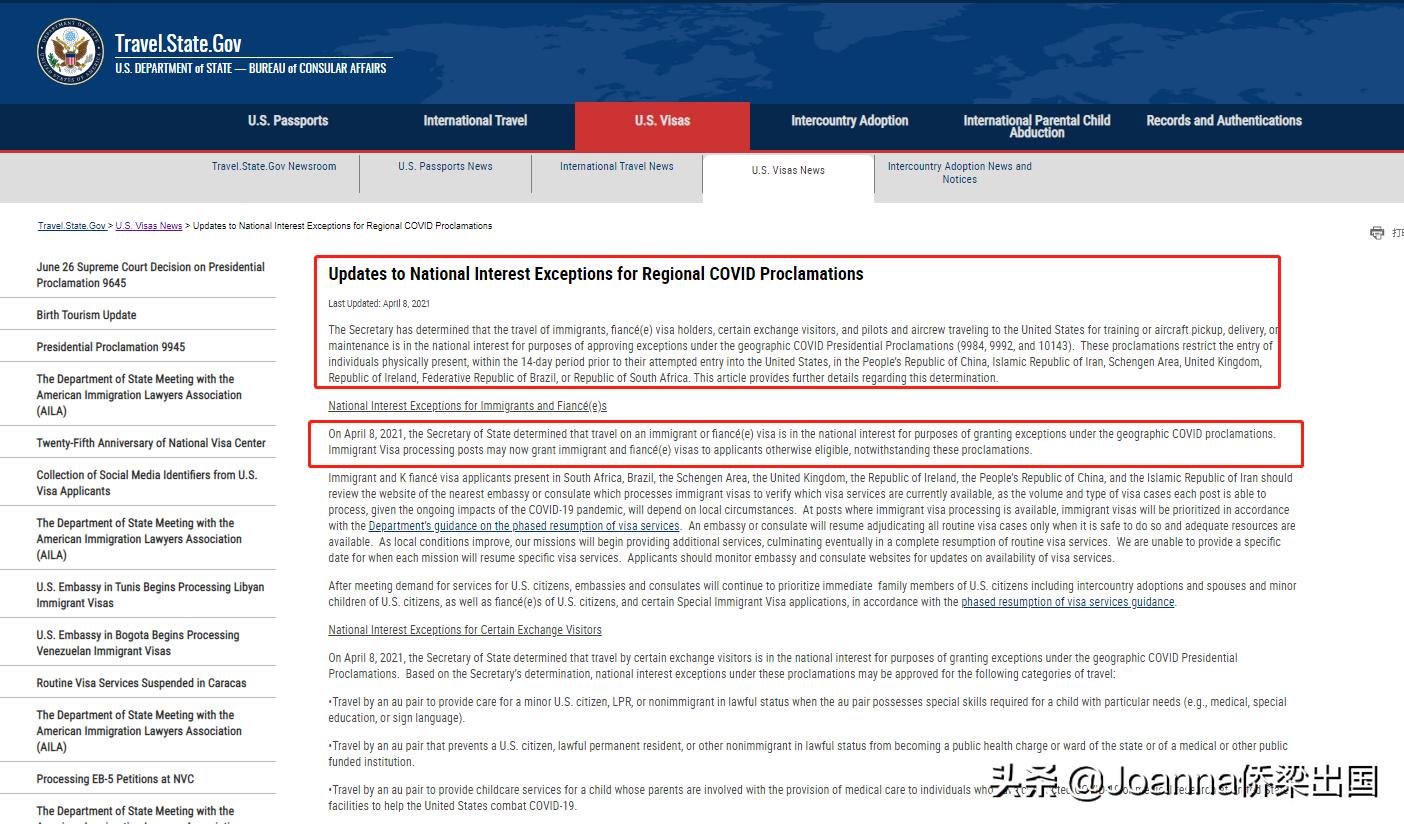A detailed screenshot of the U.S. government website, "travel.state.gov," captured from the "U.S. Department of State Bureau of Consular Affairs" section, showcasing various tabs and sections related to visas and travel updates. The top left of the screenshot prominently displays the website's title and logo, with the words "travel.state.gov" followed by a separating line and a title reading "U.S. Department of State Bureau of Consular Affairs." The section is adorned with an emblem featuring the Department of State symbol - an eagle holding a shield adorned with stars and stripes, and clutched in its talons are arrows and an olive branch, representing peace and war.

A blue banner spans the top of the webpage, subtly decorated with a faint outline of the globe's continents. Below this banner are navigational tabs that allow visitors to explore different areas such as "U.S. Passports," "International Travel," "Intercountry Adoption," "International Parental Child Abduction," "Records," and "Authentications." "U.S. Visas" is the selected tab, showing it as the active section. Directly beneath these, additional tabs offer access to news sections: "travel.state.gov newsroom," "U.S. Passport News," "International Travel News," "U.S. Visa News," and "Intercountry Adoption News and Notices."

Highlighted on the webpage is an article titled, "Updates to National Interest Exceptions for Regional COVID Proclamations," followed by extensive text detailing the updates. 

On the left sidebar, a list of additional articles or sections are visible, including headlines such as "Birth Tourism Update," "U.S. Embassy in Tunis Begins Processing Libyan Immigrant Visas," and "Processing EB-5 Petitions at NBC." 

The bottom right corner of the screenshot bears a watermark in an unidentified foreign script, which appears to be either Korean, Chinese, or Japanese, with the text, "at Johan."